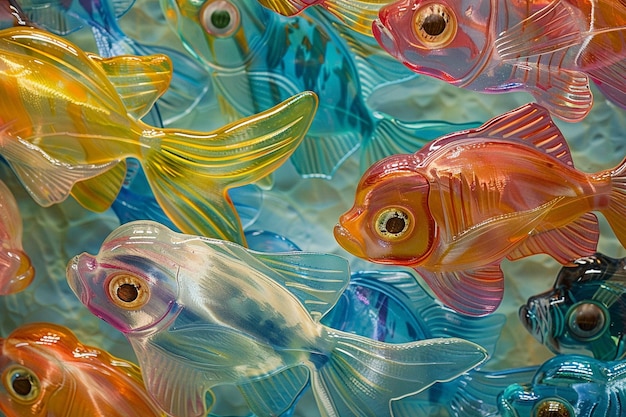This photograph captures a dense, overlapping array of goldfish figurines, which are likely made of plastic or a similar material. Each figure exhibits a uniform size and shape, characterized by realistic-looking, silvery eyes with black pupils and bulbous protruding mouths. The fish display a vibrant spectrum of colors, ranging from pale yellow, translucent shades, and various hues of blue, to more vivid orangey-red and reddish-purple tones. The camera's close-up focus and side angle allow only one eye of each figurine to be visible, enhancing their lifelike appearance. The composition reveals a layered, almost abstract arrangement with fish appearing partially in some of the cropped frame's quadrants, creating an impression of endless, overlapping fish forms. The background seamlessly blends with the figurines, amplifying the visual density and intricate detailing of the scene.